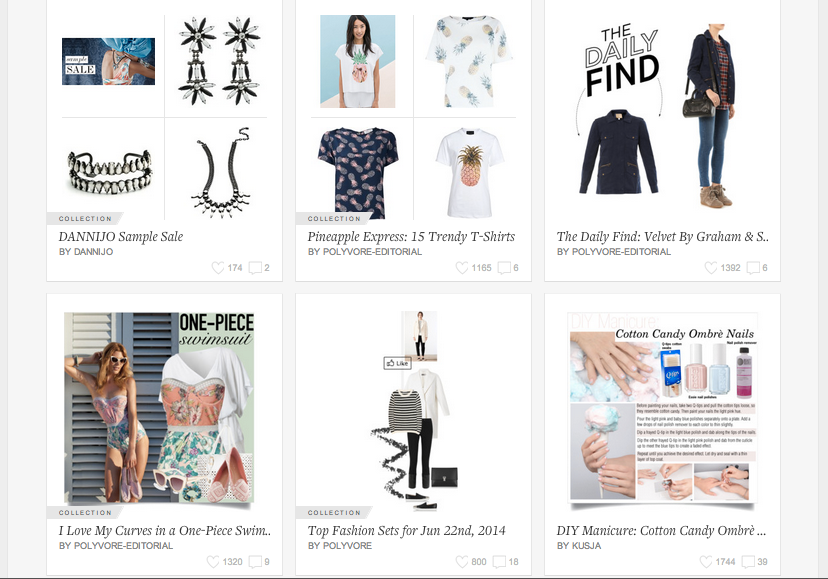This digital collage showcases a vibrant selection of fashion and beauty items. Featured prominently are images of models and various clothing pieces, including trendy T-shirts, one of which sports a playful pineapple graphic. Highlighted is a stylish ensemble featuring a woman dressed in tight denim skinny jeans paired with brown boots, a black purse, a black jacket, and a flannel shirt underneath. 

Also showcased is a detailed DIY manicure, demonstrating a cotton candy ombre design on pastel blue and pastel orange nails. The manicure process is illustrated with close-up shots of hands, cotton candy in shades of blue and yellow, q-tips, and nail polish remover. 

On the left, there is an advertisement collage for a one-piece swimsuit collection by Holly Boar, celebrating body positivity with the tagline "I Love My Curves in a One Piece Swim." The collection reflects a polished editorial style.

Completing the collage is a chic pair of sunglasses, adding a touch of sophistication to the overall fashionable theme.